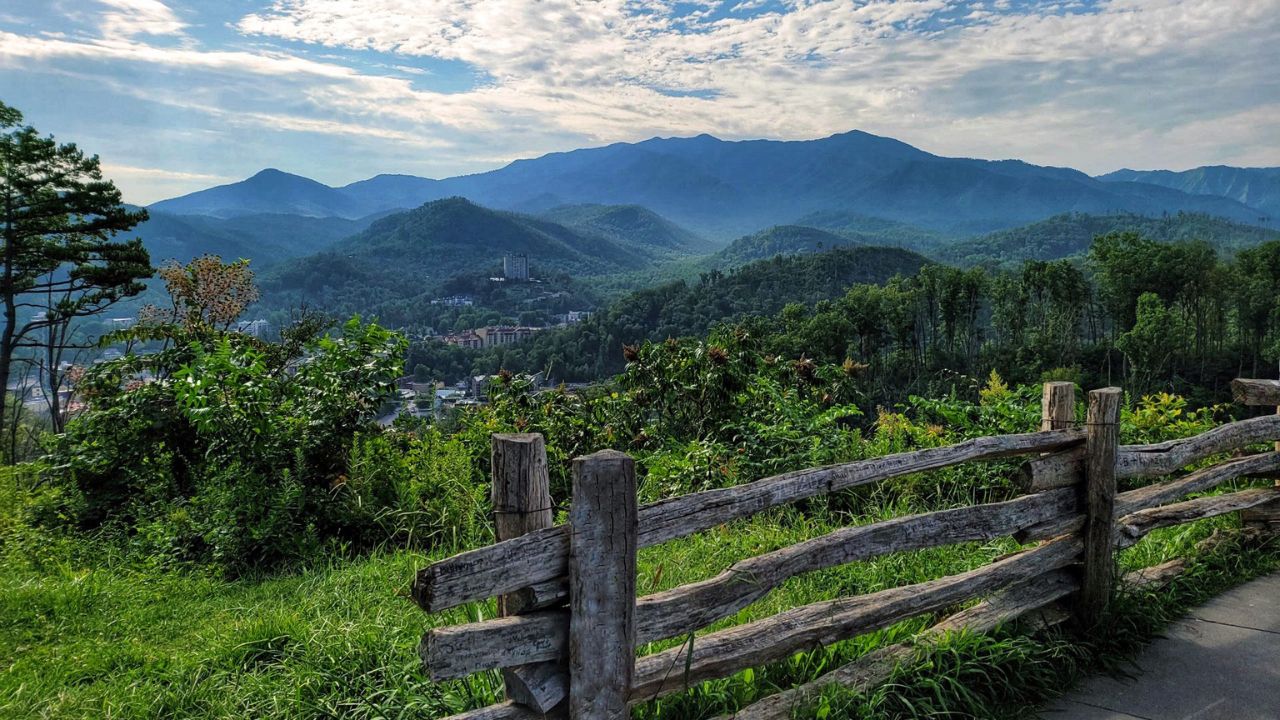The photograph captures a breathtaking nature scene from a higher elevation, looking out over a verdant valley that extends into a distant view of rolling and steep green hills, ultimately merging into dark blue-to-green mountains. The sky above is a picturesque blend of white clouds and blue, enhancing the serenity of the landscape. In the foreground, a weathered wooden post and rail fence extends from the right of the image towards the left, approximately two-thirds of the way, partially obscuring the overgrown greenery teeming with lush green weeds, white and yellow flowers, and various bushes. A portion of a sidewalk appears at the bottom right corner of the photograph. Beyond the fence, the valley overlooks a spread of indistinct buildings, suggesting a cityscape with several homes nestled amidst the greenery. The overall scene is a vibrant mix of large green and some brown trees, providing a stark contrast to the man-made structures farther away. There are no people, animals, or text visible in the photograph, allowing the viewer to fully absorb the natural beauty and tranquility of this landscape.